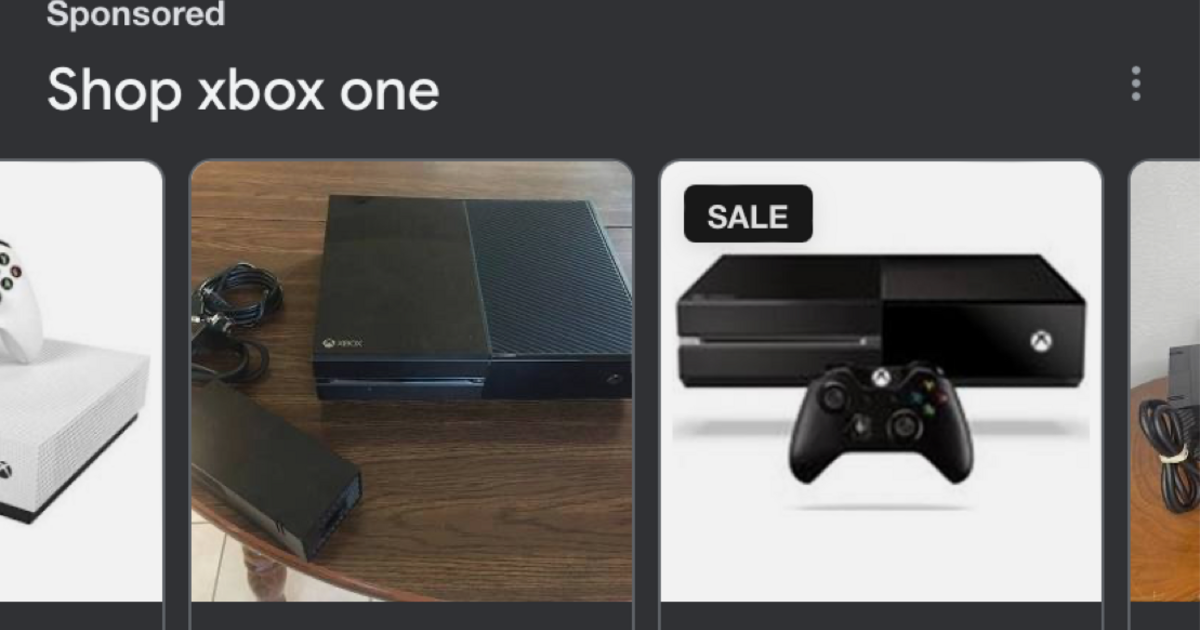The image is a screenshot with a predominantly black background, which is thicker at the top and bottom and thinner along the sides between the images. The sides display only half of the images, making them appear cut off. At the top of the image, white text reads "Sponsored" with a capital 'S'. Below that, a larger print states "Shop Xbox One," with 'S' capitalized. Toward the right side, three vertical dots in a whitish-gray color are visible.

The central section contains four images arranged vertically. The first image, partially visible, appears to show a video game console with a white body and gray trim, accompanied by a remote. The second panel features a brown wooden round table with a black Xbox gaming system and a matching black controller with some wiring visible. The third panel displays a white background with an advertisement for an Xbox video game, marked with the letter 'X' and the word "Sale" indicated at the top in white print. The final image depicts a table with part of a box, some wiring, and a rubber band.